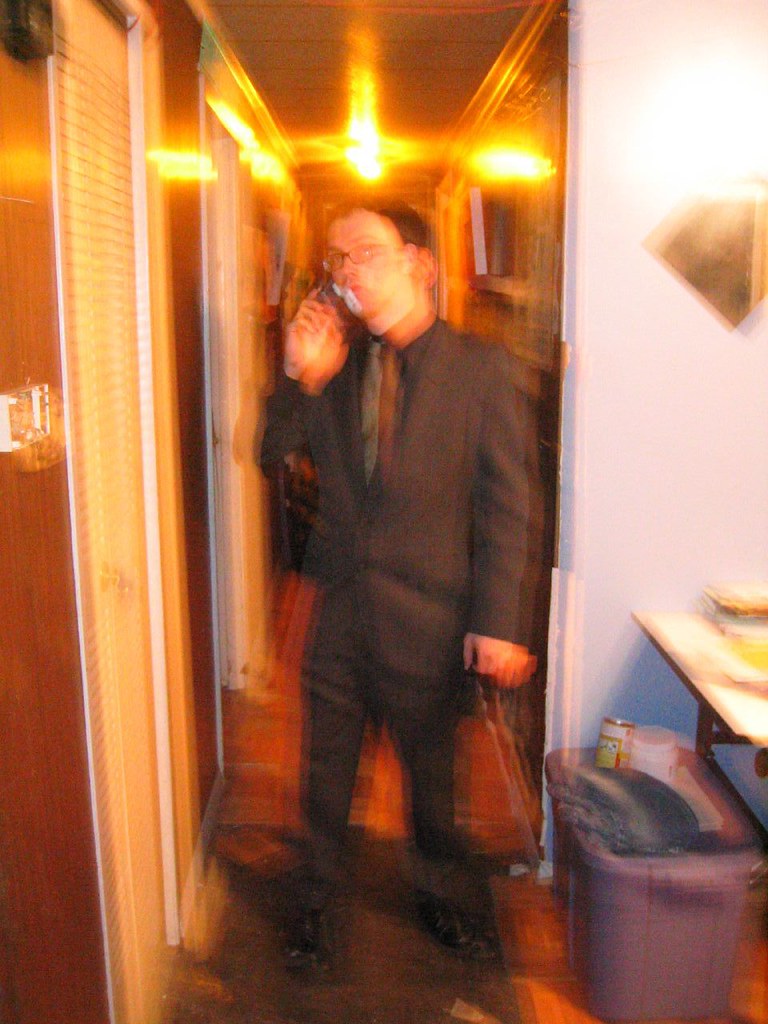The image portrays a blurry, real-life photograph of a man, likely in his late 20s or early 30s, standing in a hallway. He is dressed in a dark gray suit paired with a dark gray tie, along with black dress shoes. The man, light-skinned and wearing glasses, has short, curly black hair. In his left hand, he holds a tanned leather bag, while his right hand holds a smartphone to his ear. Above him, an orangish-yellow light casts a warm glow over the scene.

To his left, there is a door with blinds, leading to a small closet with a tan door. On his right, there's a beige table with dark brown legs, cluttered with various items including a shirt, a white canister (possibly drink powder like creatine), and a can of Chef Boyardee. Below the table is a purple storage tub, similar to those found at Walmart. The flooring appears orangish, likely due to the overhead lighting, and the hallway features a mix of light blue and dark chocolate brown walls. The image has an RGB effect, giving it a double-image appearance and adding to its overall blur.